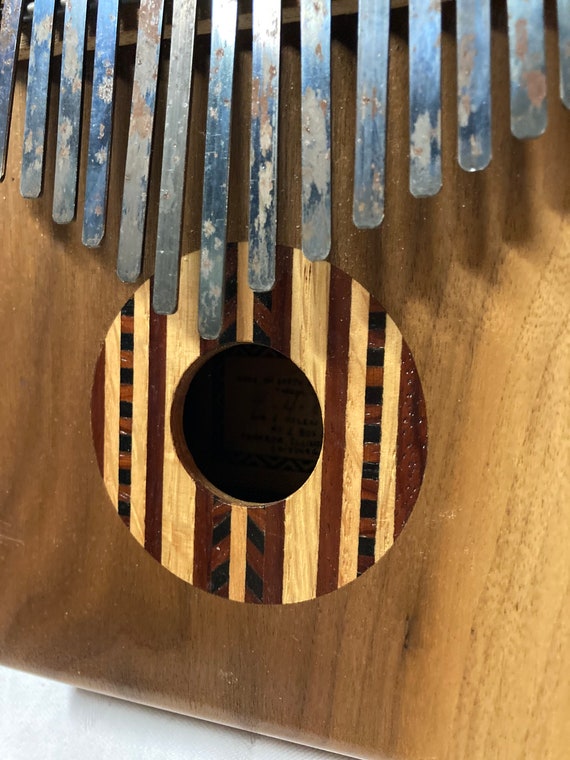The photograph depicts a handcrafted wooden musical instrument, likely a prototype or an unfamiliar variant. The body of the instrument is largely square with a prominent circular cutout at its center, featuring wood of varied grains—contrast is given by lighter and darker vertical stripes within the cutout. The primary structure is made of wood, which appears weathered and has seen some use.

Located above the circular hole, an array of rectangular metal prongs forms a fan-like arrangement. These prongs vary in length, shorter on the left, increasing towards the middle, and then shorter again towards the right. They exhibit signs of wear, with some parts retaining a shiny metallic sheen while others appear duller, possibly tarnished or slightly rusted. These metal parts could serve as keys or tines, likely being the source of sound, whether played by striking or plucking.

This instrument appears to be designed to be held either by hand or against the body, hinting at a percussive or finger-stroked playing method. The overall aesthetic and construction suggest it could be an early or experimental design of a familiar type of musical instrument, characterized by its distinctive acoustic opening and the unique arrangement of metallic tines.